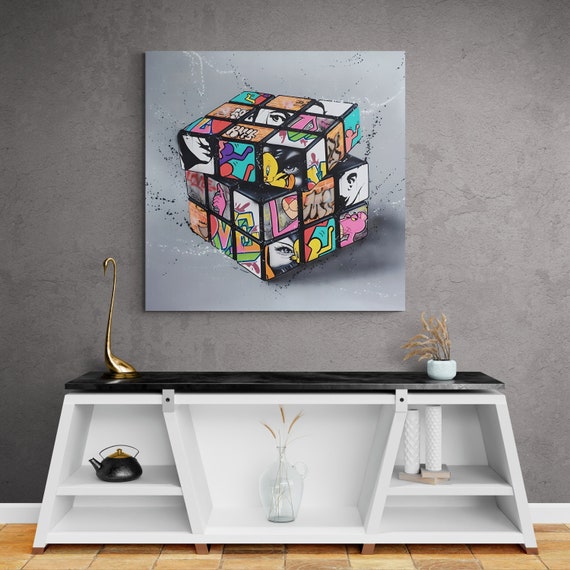The photo captures a stylish interior space featuring an art piece and a decorative white table pushed against a gray, concrete-like wall. The focal point of the image is a large painting of a partially scrambled Rubik's Cube adorned with iconic cartoon characters, including Tweety Bird and the Pink Panther, interspersed with black and white splotches and letters that seem to spell “V” and “E,” possibly hinting at the word "love." Below the painting is a sleek white table with a black top. The table holds a variety of decorative items: a golden swan figurine perched elegantly on the top, a white vase, and a black tea kettle. The open shelves of the table reveal additional vases, including a clear jar with a handle that contains some green plants. The floor in the image is wooden, contributing to the room's modern yet cozy ambiance.